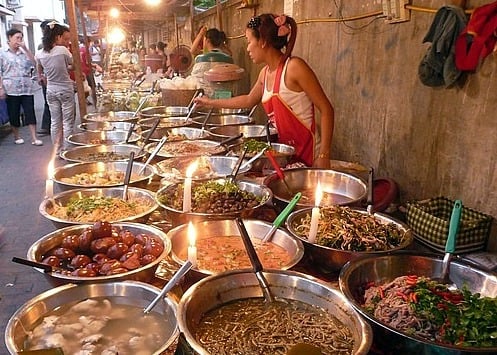In this vivid depiction of an Asian street market, the focal point is a thin woman with black hair tied into a ponytail adorned with a pink bow and a black headband. She is dressed in a white tank top and a red apron, and stands behind a large, long table laden with rows of big silver bowls, each equipped with its own ladle. The bowls are filled with a variety of foods, including broths, soups, stews, noodles, rice, and different types of meat. Some of the bowls are accompanied by white lit candles, adding to the vibrant scene. In the background, other shoppers and vendors can be seen, enhancing the bustling atmosphere of the market. The scene captures the essence of a lively culinary setting, with people examining the dishes, trying to decide what to savor amidst the myriad of options.